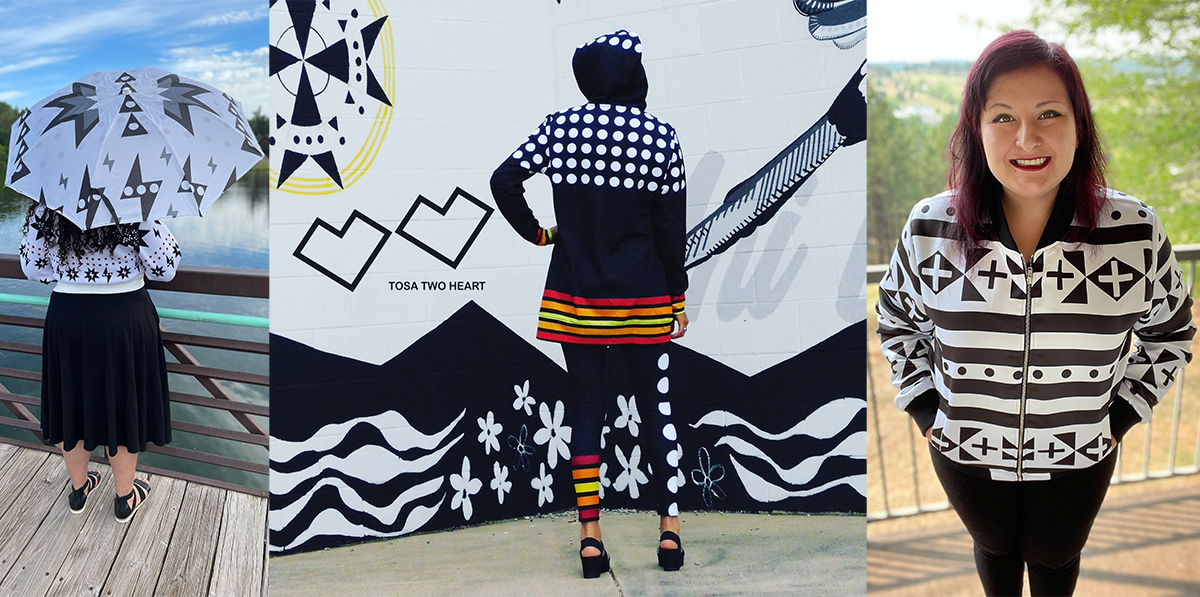The triptych features three women in striking black and white garments, presumably designed by Tosa Two Heart. The left panel depicts a woman standing on a wooden dock overlooking a lake, dressed in a black mid-length skirt, black sandals, and a black and white patterned sweater. She holds a black and white umbrella that mirrors the design of her sweater and has dark, curly hair. The central panel showcases a large black and white mural with geometric shapes and the name "Tosa Two Heart." In front of this mural, another woman stands on a concrete surface. She wears a black hooded jacket and pants, both adorned with white polka dots, featuring red, orange, and green stripes at the bottom of the jacket. The right panel presents a smiling woman facing the camera, clad in a black and white zip-up jacket with plus and minus signs. She sports black leggings and dark, reddish-black hair.